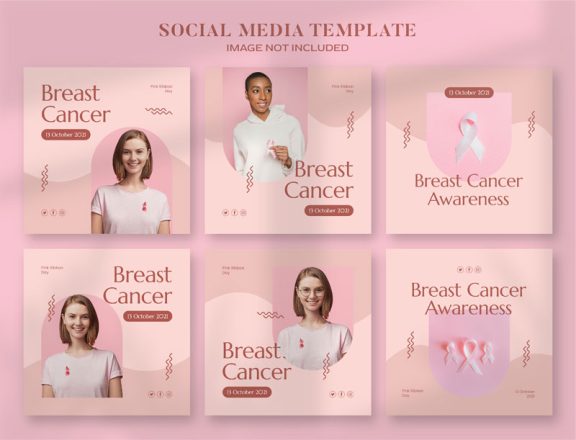The image is framed in a slightly horizontal rectangular shape and features a pink background with varying shades. The pink hue fluctuates, especially noticeable at the top and center of the background. The top of the image contains the text "Social Media Template, Image Not Included." Below this text, there are two rows, each consisting of three square images focused on breast cancer themes. Of the six templates, four include images of women, while two are centered around breast cancer ribbons. One prominently displays a single pink breast cancer ribbon, and the other features three such ribbons. The legible text on the templates reads phrases like "Breast Cancer" and "Breast Cancer Awareness," although other smaller text remains illegible.